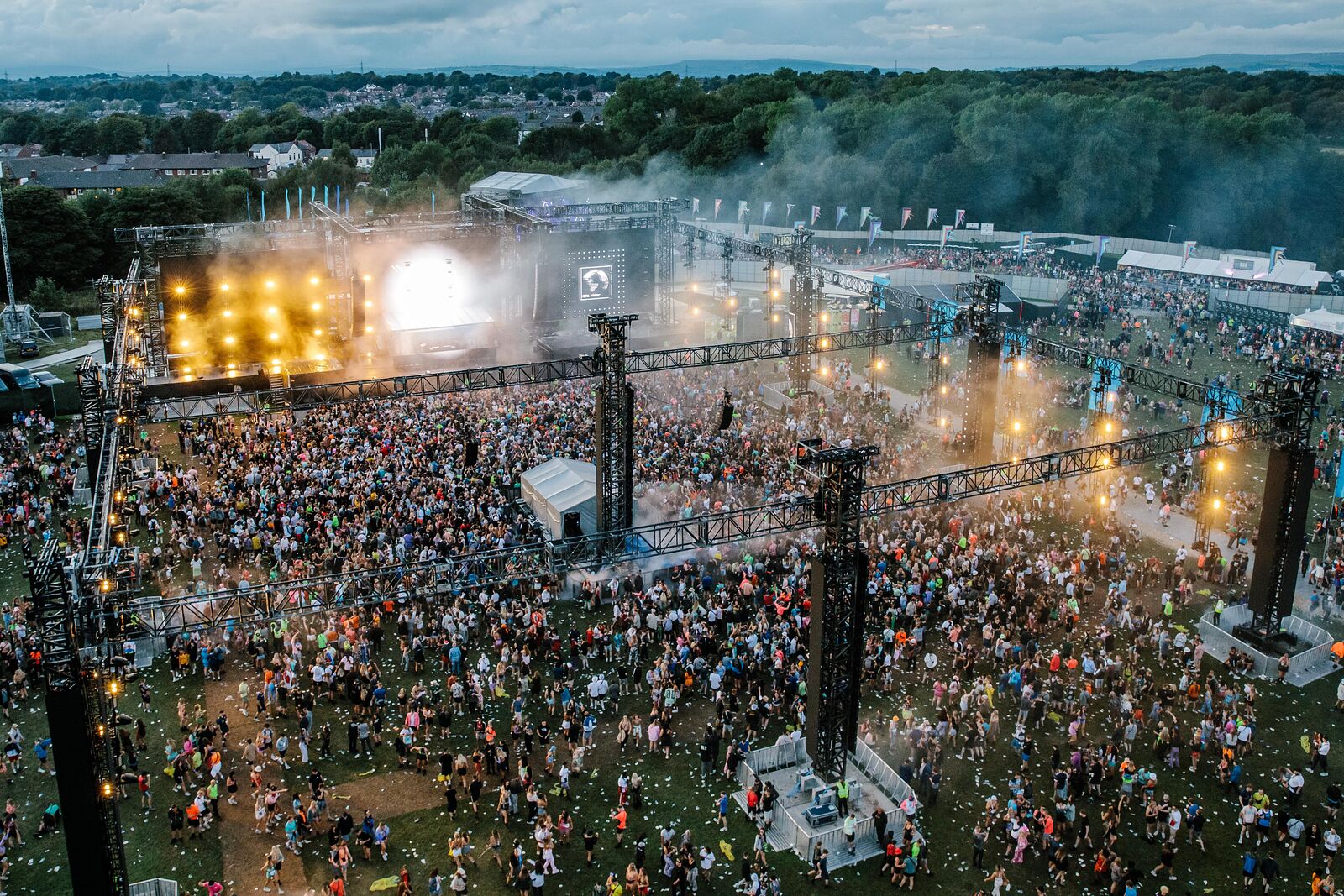This extensive aerial photograph captures an outdoor concert in a large, grassy venue crowded with thousands of attendees. The image, taken from above, showcases the stage situated near the top left corner, draped in stage fog from fog machines. Bright yellow spotlights illuminate the left side of the stage, which is framed by black metal scaffolding forming a square and further adorned with yellow lights. The ground below is strewn with what appears to be either trash or confetti, contributing to the chaotic yet festive atmosphere. In the distance to the right, additional gathering areas are visible, marked by numerous tents and hanging flags. The backdrop features lush green trees and a sky filled with white and gray clouds, with distant buildings peeking through, completing this vibrant and dynamic scene.